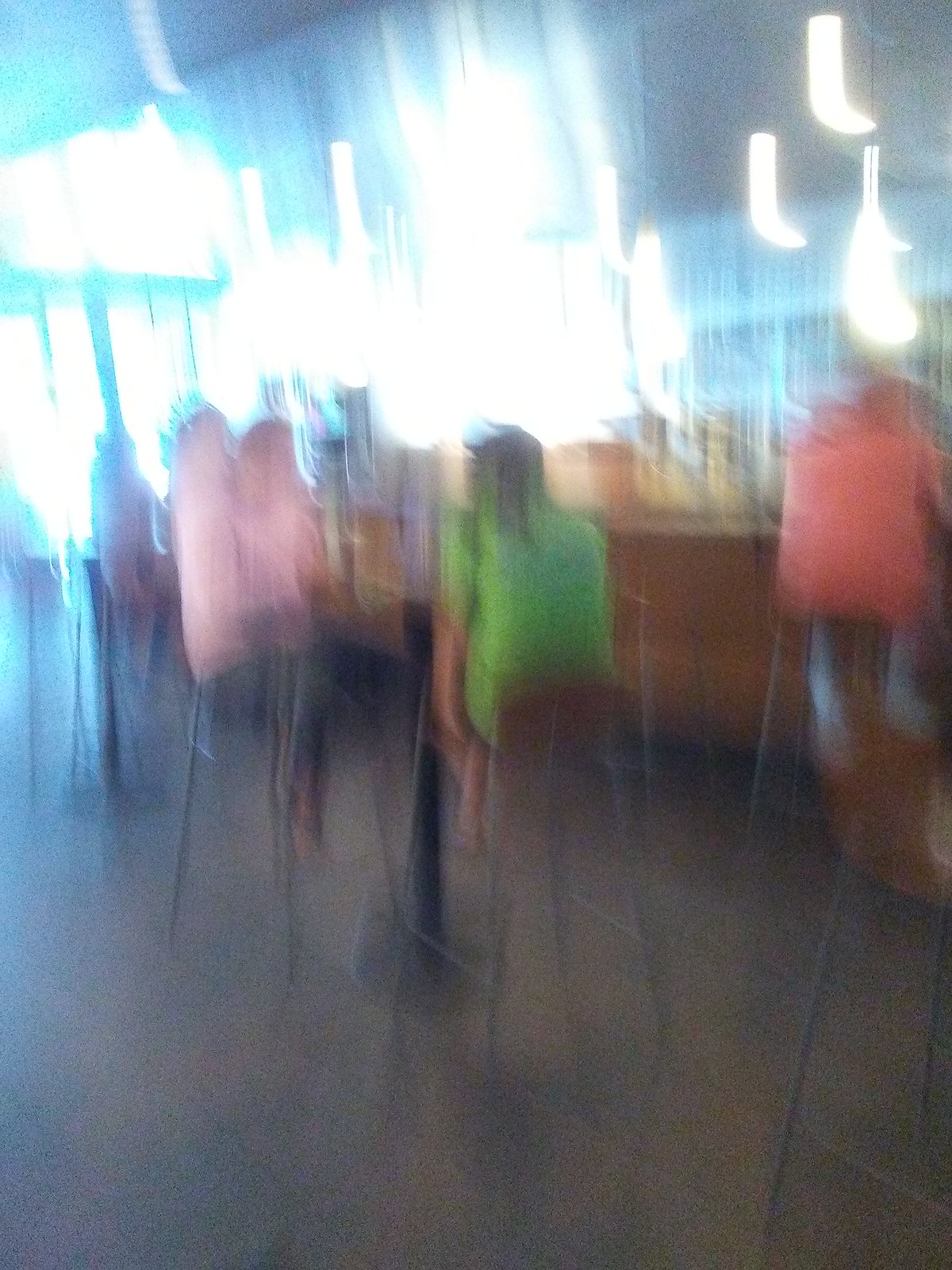This portrait-oriented, very blurry photograph captures the interior of a bar or coffee shop. The image is heavily streaked and distorted, rendering most details indistinct. A wooden bar counter stretches across the scene, populated with blurred bottles at the back and blurred hanging lights above. To the far right, a figure in a red shirt or anorak and blue pants sits at the counter on a bar stool. Centered in the foreground is a tall, pedestal table with elevated chairs, where two women are seated. The woman with her back to us wears a green top or dress, while her companion, seated opposite, sports a pink shirt. The background is brightly illuminated by daylight streaming through large, glass windows or doors on the left, casting a washed-out, luminous effect.